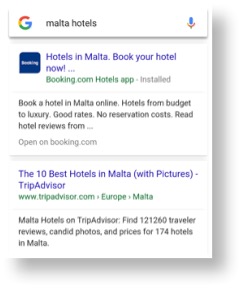A screenshot of a Google search results page for "Malta hotels" shows various information sources related to booking accommodations in Malta. Directly beneath the search bar, there is a snippet featuring a small square image next to the text "Hotels in Malta. Book your hotel now" in blue font. Below this, a green link reads "Booking.com Hotels App," accompanied by the word "Installed" in gray. Further down, a gray text line suggests "Book a hotel in Malta online. Hotels from budget to luxury. Good rates, no reservation costs. Read hotel reviews from..." followed by an ellipsis. Another gray link prompts to "Open on Booking.com."

Additionally, the search results feature a blue link titled "The 10 Best Hotels in Malta - TripAdvisor," followed by a green URL: "www.tripadvisor.com › Europe › Malta." Below this, gray text indicates "Malta hotels on TripAdvisor: Find 121,260 traveler reviews, candid photos, and prices for 174 hotels in Malta." This is the end of the visual content in the screenshot.